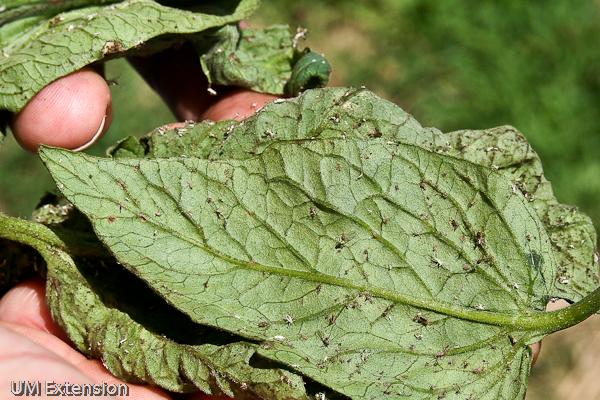In this close-up photograph, two hands, presumably of a Caucasian individual, are holding a couple of leaves against a blurred, green background, suggesting an outdoors setting. The leaves are prominently featured in the center of the image, showing intricate details such as veins, dirt, and numerous black and white spots indicative of a possible fungal disease or tiny bug infestation. One of the leaves appears to be flipped over, exposing its underside covered in these abnormal markings. The words "UM Extension" are visible in the lower right-hand corner of the photograph, hinting at an affiliation with an academic or agricultural extension program. The overall scene is bathed in sunlight, enhancing the detailed textures and the focus on the leaf's condition.